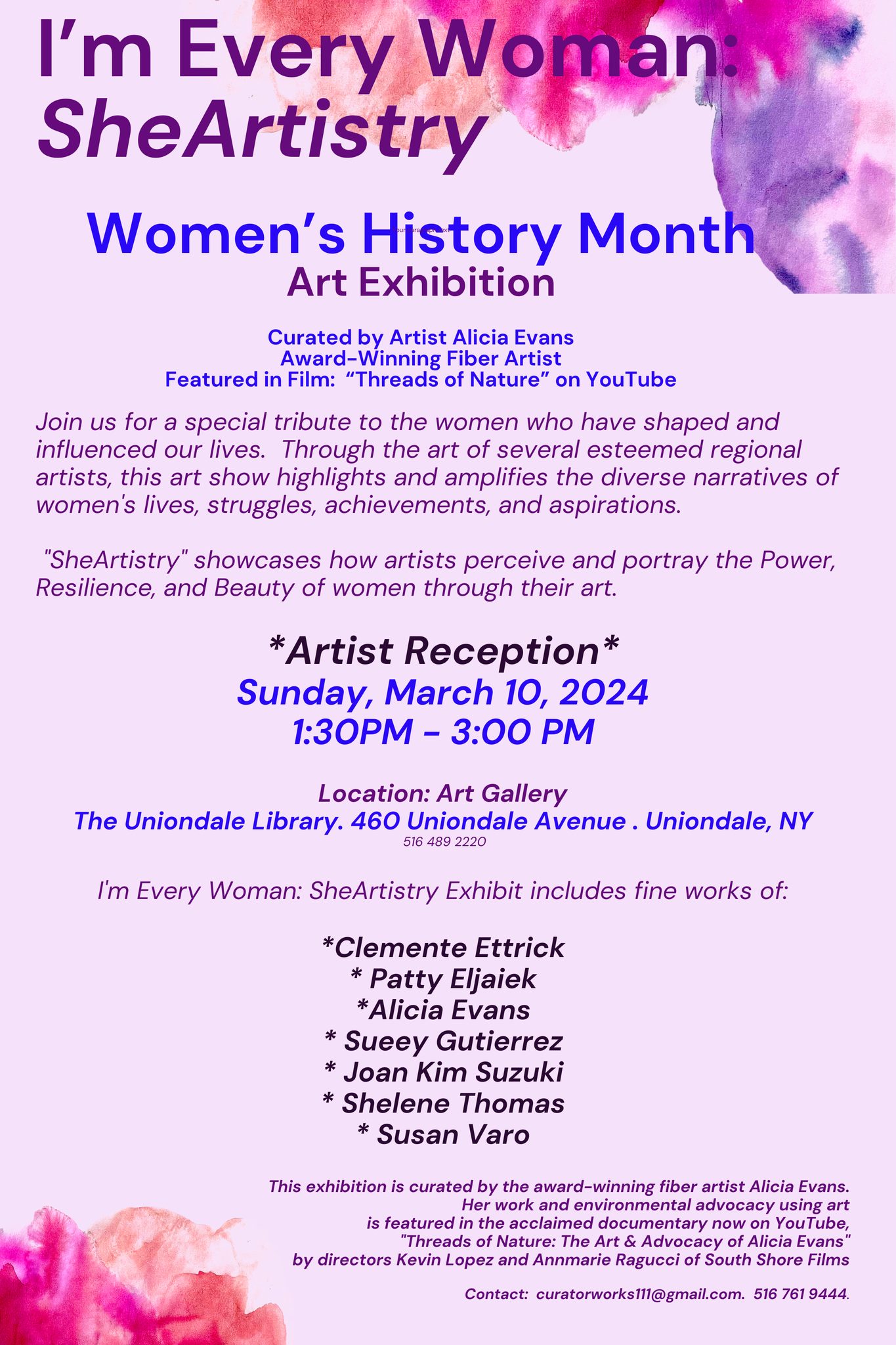The image showcases a digital screenshot of a flyer, predominantly colored in light purple with accents of dark purple, dark blue, and hints of pink, orange, red, and blue. This flyer advertises an art exhibition titled "I'm Every Woman She Artistry" in honor of Women's History Month. Created by award-winning fiber artist Alicia Evans, who is also featured in the YouTube film "Threads of Nature," the exhibition will be held on Sunday, March 10, 2024, from 1:30 to 3:00 p.m. at the Art Gallery in the Uniondale Library, located at 460 Uniondale Avenue, Uniondale, New York. The event includes an artist recognition ceremony and showcases the works of artists Clementine Itrick, Patti Eliajack, Alicia Evans, Sue Katerios, Joan Kamsuzuki, Chalene Thomas, and Susan Vero. Additionally, the flyer features an illustration of flowers, emphasizing the artistic theme of the event.